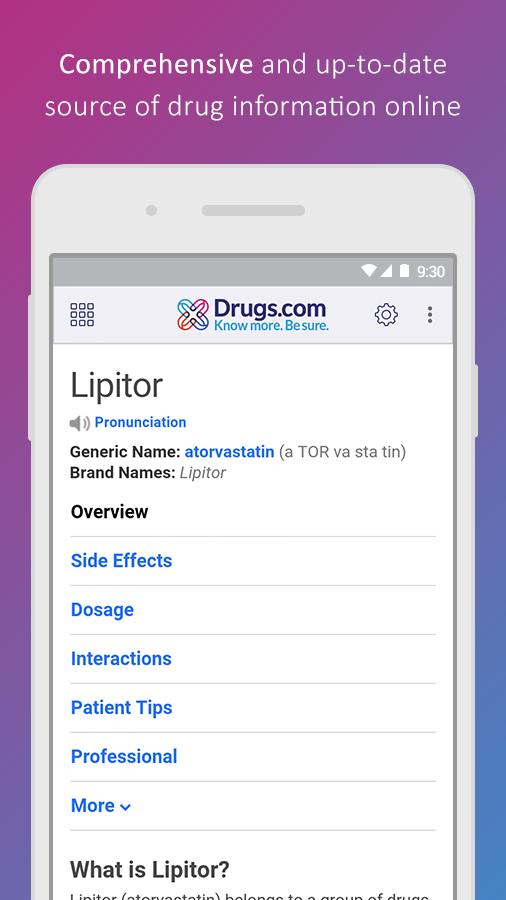The advertisement showcases the Drugs.com platform on a gradient background that transitions from a light purple at the top left to a darker purple and blue towards the bottom. At the top of the ad, bold white letters announce: "Comprehensive and up-to-date source of drug information online." Below this statement, a white iPad dominates the visual center. On the iPad's screen, the Drugs.com interface is prominently displayed, featuring the Drugs.com logo at the center, accompanied by the reassuring message "No more be sure" in light blue text underneath.

The iPad screen is specifically open to the drug Lipitor's page. A speaker icon appears below the drug name, indicating that users can click to hear the pronunciation, which is accompanied by the word "Pronunciation" in light blue text. The page also provides both the generic and brand names of Lipitor. In the center, several categories are visible, including overviews, side effects, dosage, interactions, patient tips, and professional information; the "More" category features a drop-down box.

At the bottom of the screen, the text "What is Lipitor?" can be partially seen, hinting at more detailed information available further down the page. The image is cropped before showing the entirety of this section.